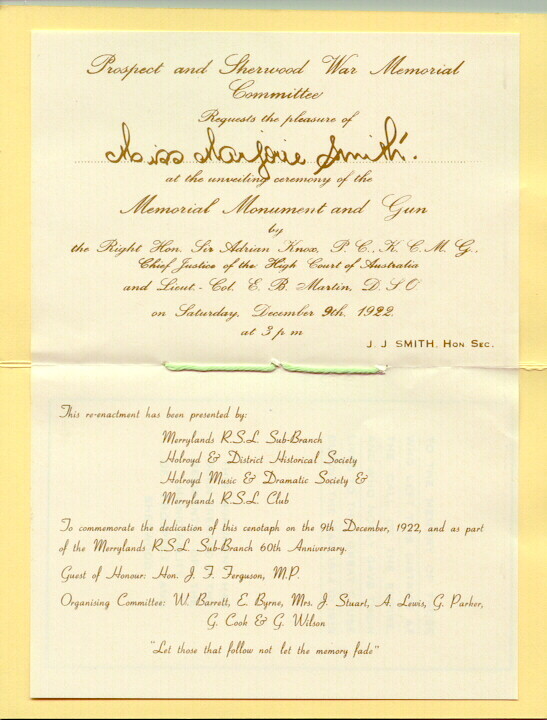The image shows a single piece of crinkled paper, positioned centrally and occupying most of the frame. The paper is light yellow and appears to be affixed to or lined with a yellowish background. The text on the paper is written in an elegant cursive script in brown ink. At the top, it reads "Prospect and Sherwood War Memorial Committee requests the pleasure of," followed by a partially legible handwritten name, the last name being Smith. The text continues with an invitation to the unveiling ceremony of the Memorial Monument and Gun, officiated by the Right Honorable Sir Adrian Ngo, Chief Justice of the High Court of Australia, and Lieutenant Colonel E.B. Martin. The event is scheduled for Saturday, December 9th, 1922, at 3 p.m. The reenactment is presented by Maryland's RSL Subbranch, Holroyd and District Historical Society, Holroyd Music and Dramatic Society, and Maryland's RSL Club to mark the dedication of the monument and to celebrate the 60th Anniversary of Maryland's RSL Subbranch. The paper also mentions the Guest of Honor, Honorable J.F. Ferguson MP, and lists the organizing committee's names. The colors in the image include shades of gray, yellow, tan, maroon, and a light green. The overall setting suggests an old, historical document related to a war memorial.